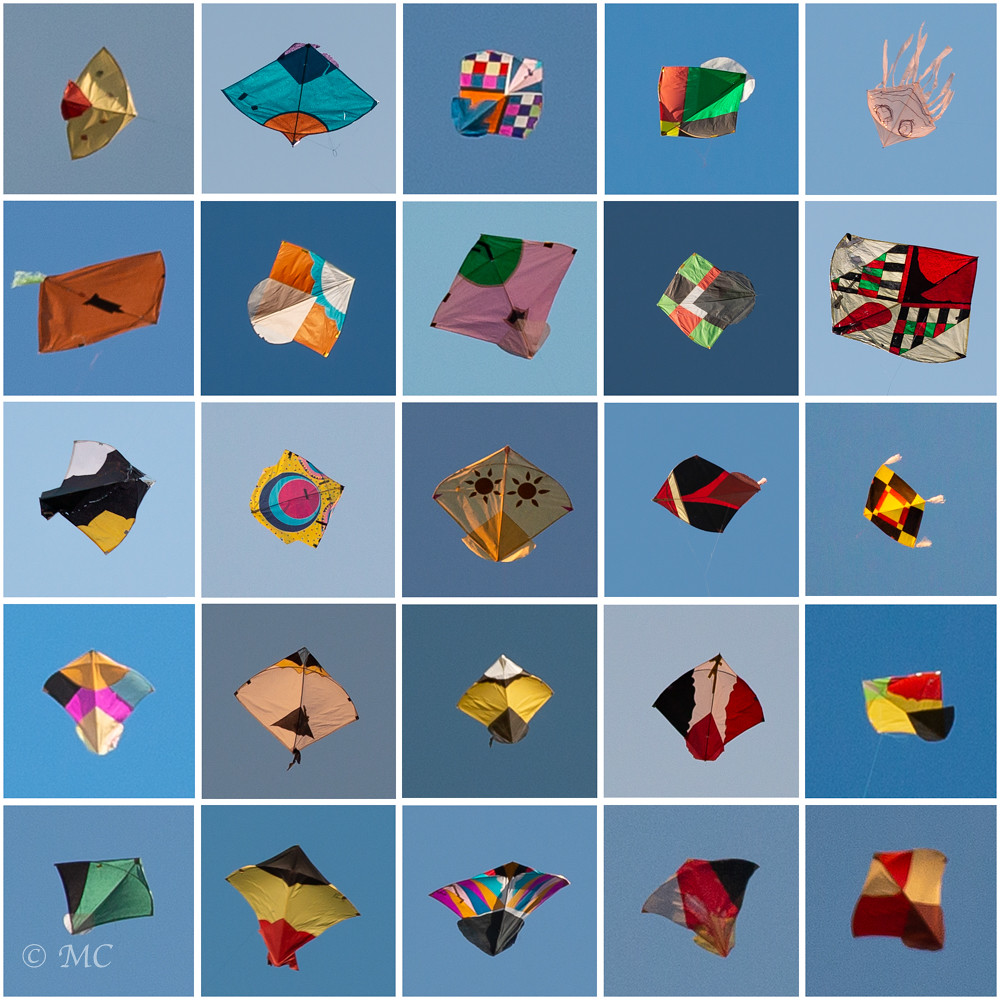The image is divided into a 5x5 grid, with a total of 25 small squares. Each square features a different kite set against a backdrop of blue sky, with some parts of the sky being darker and others lighter. The kites are a diverse array of shapes and colors, including diamonds, squares, triangles, and some with teal feathers. The colors of the kites are hugely varied, ranging from pink checkered squares to bright reds, oranges, greens, blues, browns, and even combinations like red, white, and blue. Here and there, you can spot strings still attached to the kites. Additionally, the bottom left-hand corner of the image features a circle with the letters "C" and "MC" written in white.